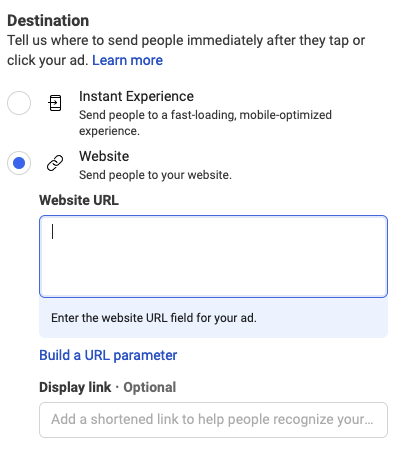This image is a detailed interface screenshot for setting the destination of an advertisement. The background is white with black text prominently displayed in the upper left corner. The first line reads "Destination" in bold text. Below it, in smaller font, the text instructs: "Tell us where to send people immediately after they tap or click your ad." To the right of this, “Learn More” is highlighted in blue.

The next section features a white circle with a light gray outline, housing a phone icon with an arrow pointing to the right, next to the label "Instant Experience." Below this, in smaller text, it explains: "Send people to a fast-loading mobile-optimized experience."

Further down, another white circle with a gray outline appears, this time containing a blue dot in the center. It is adjacent to a chain link icon and the bold black text "Website." Below this header, smaller text directs: "Send people to your website," followed by the prompt "Website URL."

Under the prompt is a large rectangular input field meant for entering the website URL, with accompanying instructions: "Enter the website URL field for your ad." Following this are options to "Build a URL Parameter" and an optional "Display Link" field, complete with another rectangle for adding a recognizable shortened link.